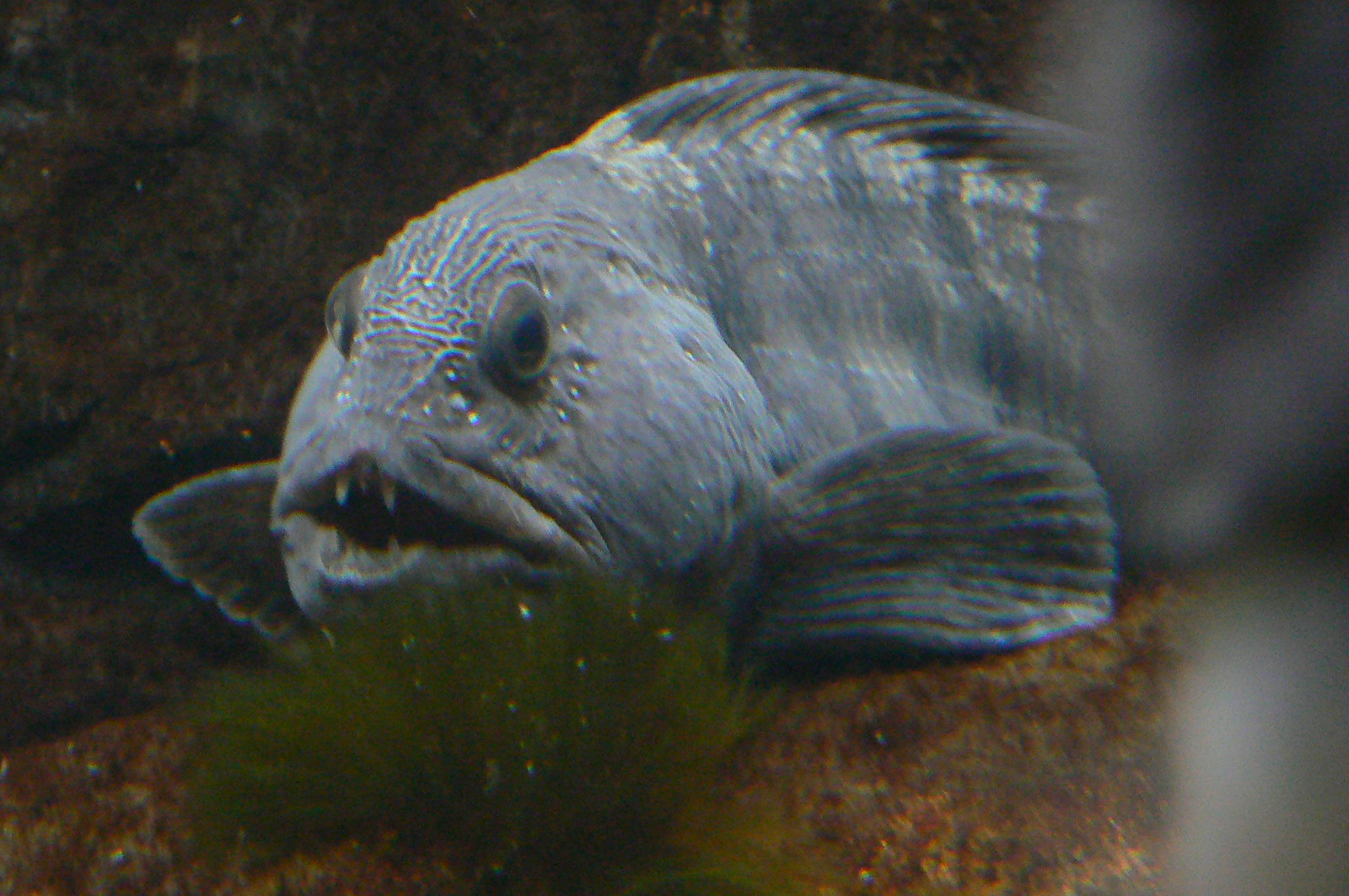This close-up image captures a unique, grayish-blue fish in what appears to be an aquarium. The fish, primarily gray with lighter splotches and darker stripes, is the focal point, positioned with its head on the left and its body extending to the right, partially cut off. Its head is slightly turned towards the viewer, revealing black, beady eyes and a somewhat open mouth with prominent fangs—two on the top and two or three on the bottom against the dark void of its mouth, giving it an angry or menacing expression. 

The backdrop features a bed of brownish stones and a noticeable green plant in the bottom left corner, characterized by thin, green strands. A blurry gray strip is visible on the right side of the image, contributing to the sense of depth. The overall scene suggests a well-maintained aquarium environment, with clear water and intentional decoration, highlighting the unique appearance of the fish and its seemingly aggressive demeanor.